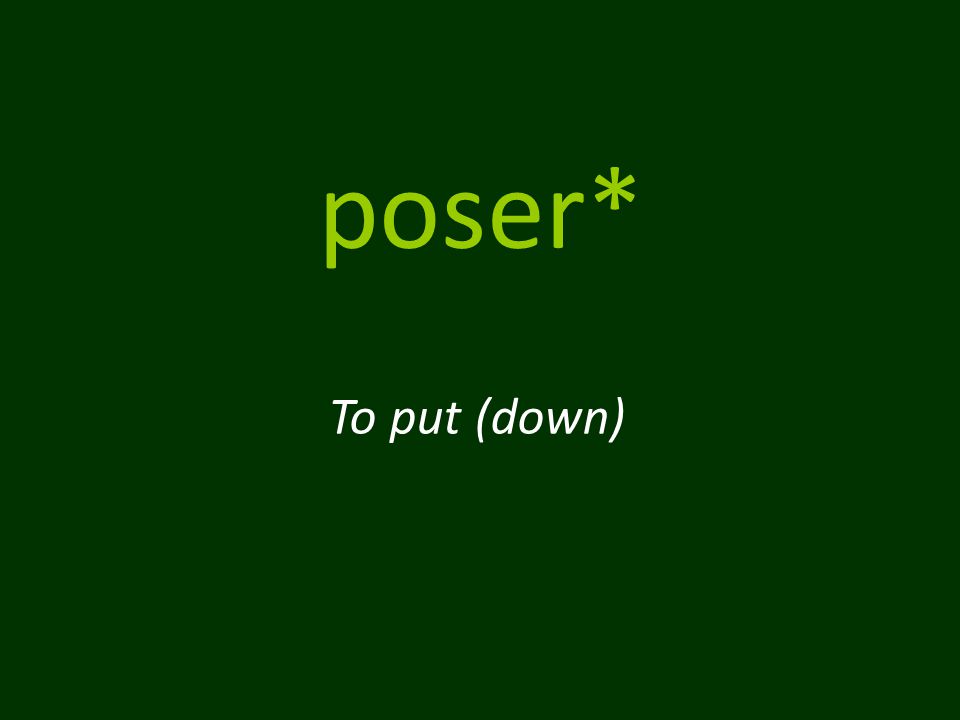The image features a large rectangular slide with a dark, forest green background resembling the color of a plant leaf. This simple design seems intended for an educational presentation. The slide's dimensions favor a slightly longer horizontal side. Centered in the upper third of the slide is a word written in a light lime green font, "poser," all in lowercase, followed by an asterisk to the upper right of the last letter. Directly beneath this, in white font, is a phrase with the word "to" capitalized, reading "TO PUT," and in parentheses directly following, the word "down." The overall appearance is minimalistic, with these two lines of text standing out sharply against the dark green backdrop.